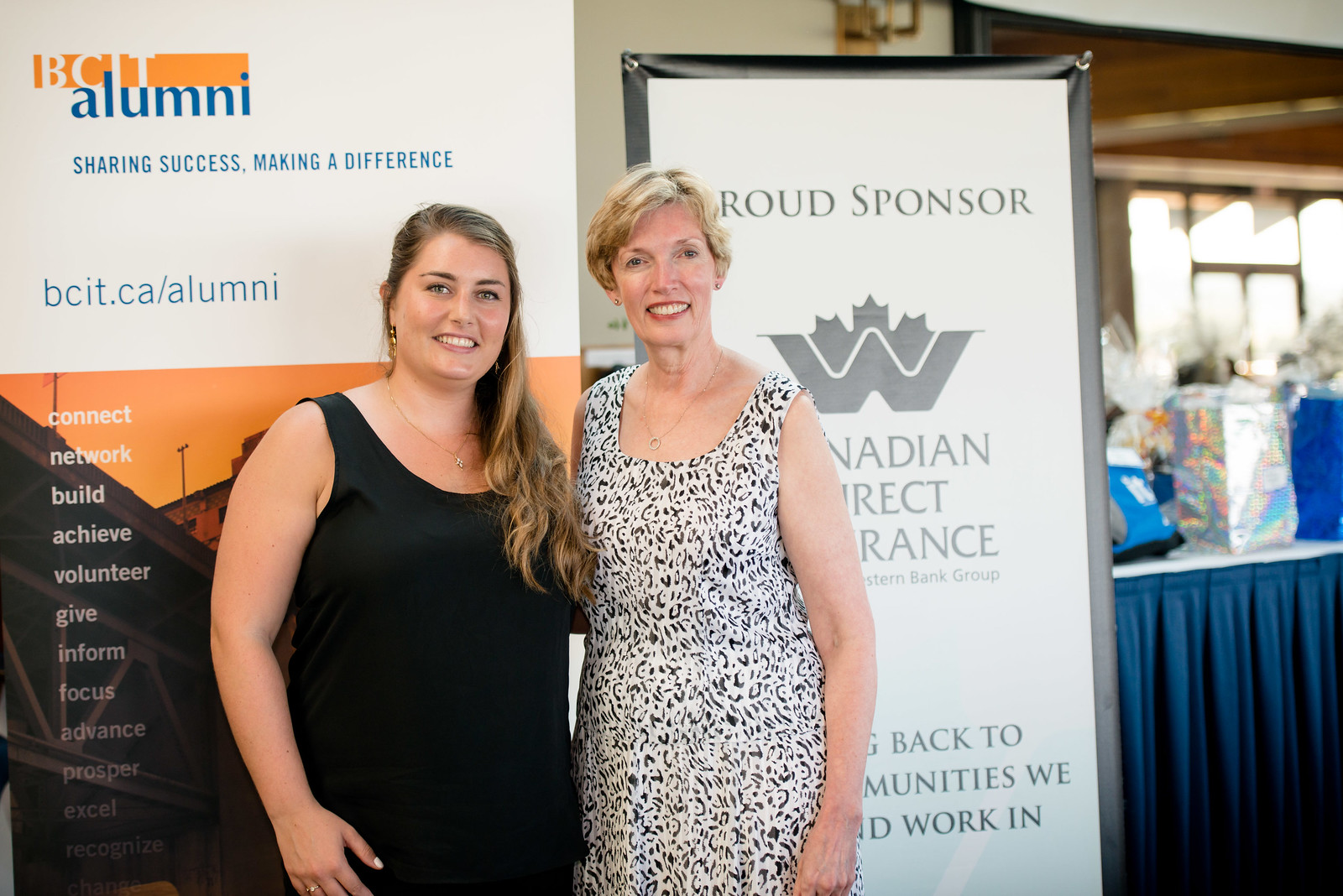This photograph depicts two white women standing in front of convention billboards. On the left is a younger woman with long, dark blonde hair that flows over her left shoulder. She is wearing a sleeveless black outfit and a necklace, smiling at the camera with her right hand near her right hip. To her right stands an older woman, possibly the younger woman's mother, wearing a white and black speckled dress. She has short blonde hair and a wide smile, with her left arm down at her side, suggesting the two might have their arms around each other. 

The background features two billboards. The one behind the younger woman reads, "BCIT Alumni: Sharing Success, Making a Difference," with additional text including a website address, "bcit.ca/alumni," and vertically arranged words like "connect," "network," "build," "achieve," and "volunteer." The billboard behind the older woman features the text, "Proud Sponsor Canadian Direct Insurance," though part of the wording is blocked by her position. 

Additional background details include a table draped with a blue curtain, situated to the right of the women, holding some items including a gift bag. Further behind them on the right, part of the convention hall can be seen, including a door, some windows, and the roof structure of the building.